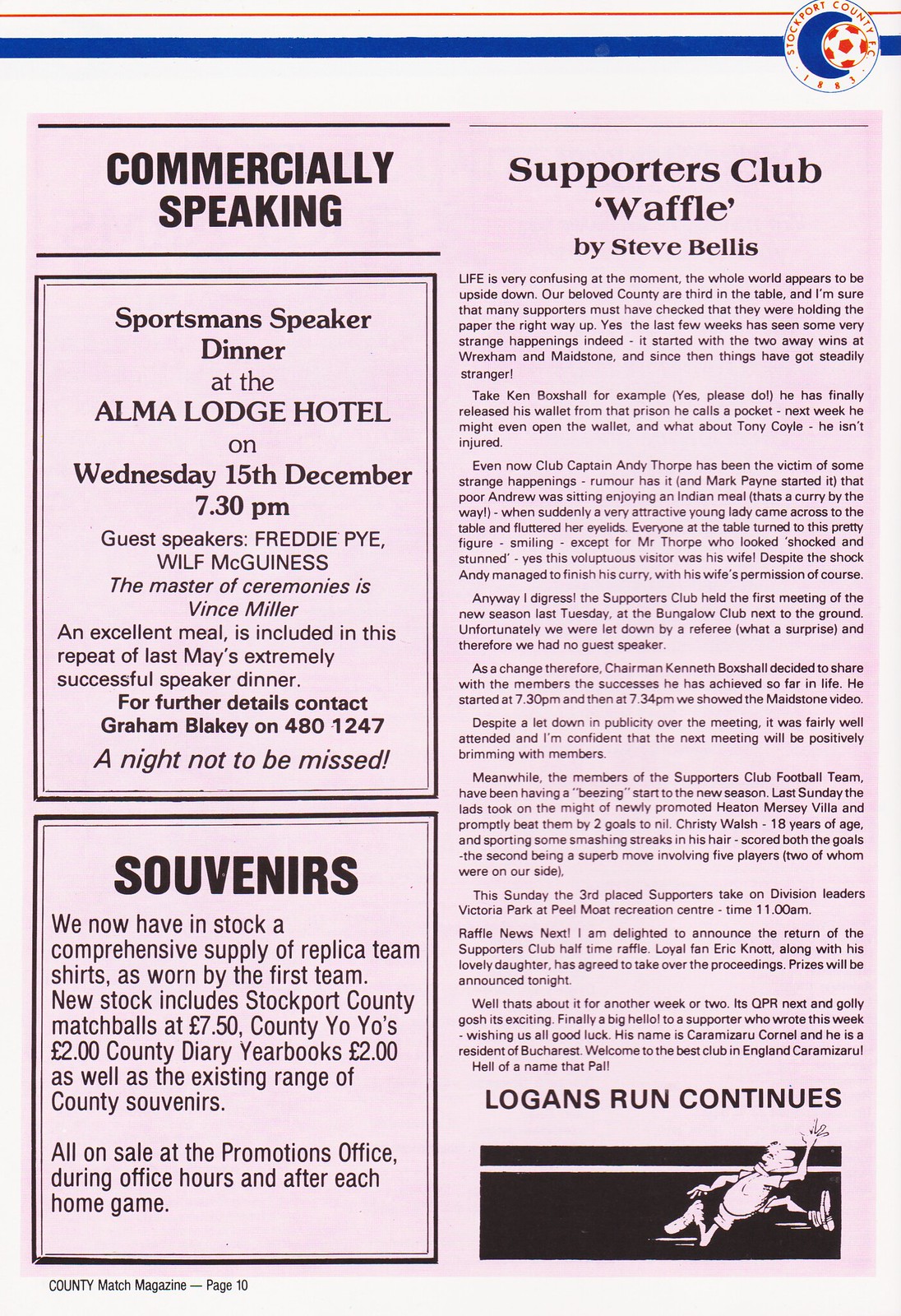This image is a color scan of a rectangular magazine page featuring an advertisement and textual sections. The page has a varied color palette with an off-white background, a thick blue band at the top, and a prominent red logo for Stockport County FC, which includes the text "Stockport County, 1883" and a red soccer ball. The left column features two boxed advertisements beneath the header "Commercially Speaking." The first box advertises a "Sportsman Speaker Dinner" at the Alma Lodge Hotel on Wednesday, December 15th, at 7:30 p.m., listing Freddie Pye and Wolf McGinnis as guest speakers, with Vince Miller as the Master of Ceremonies. The advertisement highlights that excellent meals are included and invites readers to contact Graham Blakey for further details. The second boxed section titled “Souvenirs” lists various memorabilia such as replica team shirts, Stockport County match balls priced at $7.50, County yo-yos at $2, and County yearbooks, all available at the Promotions Office during office hours and after home games.

The right column consists of a lengthy article titled "Supporters Club Waffle" by Steve Bellis. Below the article is another section titled "Logan's Run Continues," accompanied by a small drawing of a man running towards the right. The page also includes a small footer in the bottom left corner reading "County Match Magazine, page 10." The overall layout combines detailed event promotion with team memorabilia sales and editorial content, providing comprehensive coverage for Stockport County FC fans.